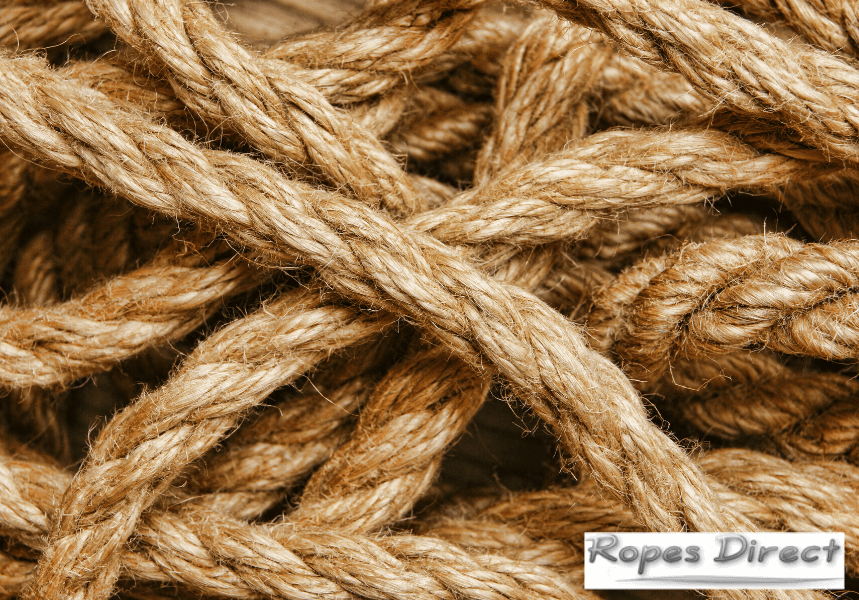The image is a highly detailed, close-up shot of a tangled mass of tannish-brown braided cloth ropes, filling the entire frame. The ropes display varying hues of brown and tan, with some braided together while others remain free and intertwined haphazardly, creating a complex and textured appearance. Fine details, such as small protruding fibers, indicate the rough texture and older material of the ropes. The lighting of the image is ambiguous, leaving it unclear whether it is illuminated by natural sunlight or artificial lighting. In the bottom right-hand corner, the phrase "Ropes Direct" is prominently displayed in a gray cartoonish font on a white rectangle, underlined by a small gray line. This label is superimposed directly on the image, providing a slight visual contrast to the chaotic scene of ropes. The overall layout of the ropes appears random and unstructured, emphasizing the natural, organic feel of the scene.